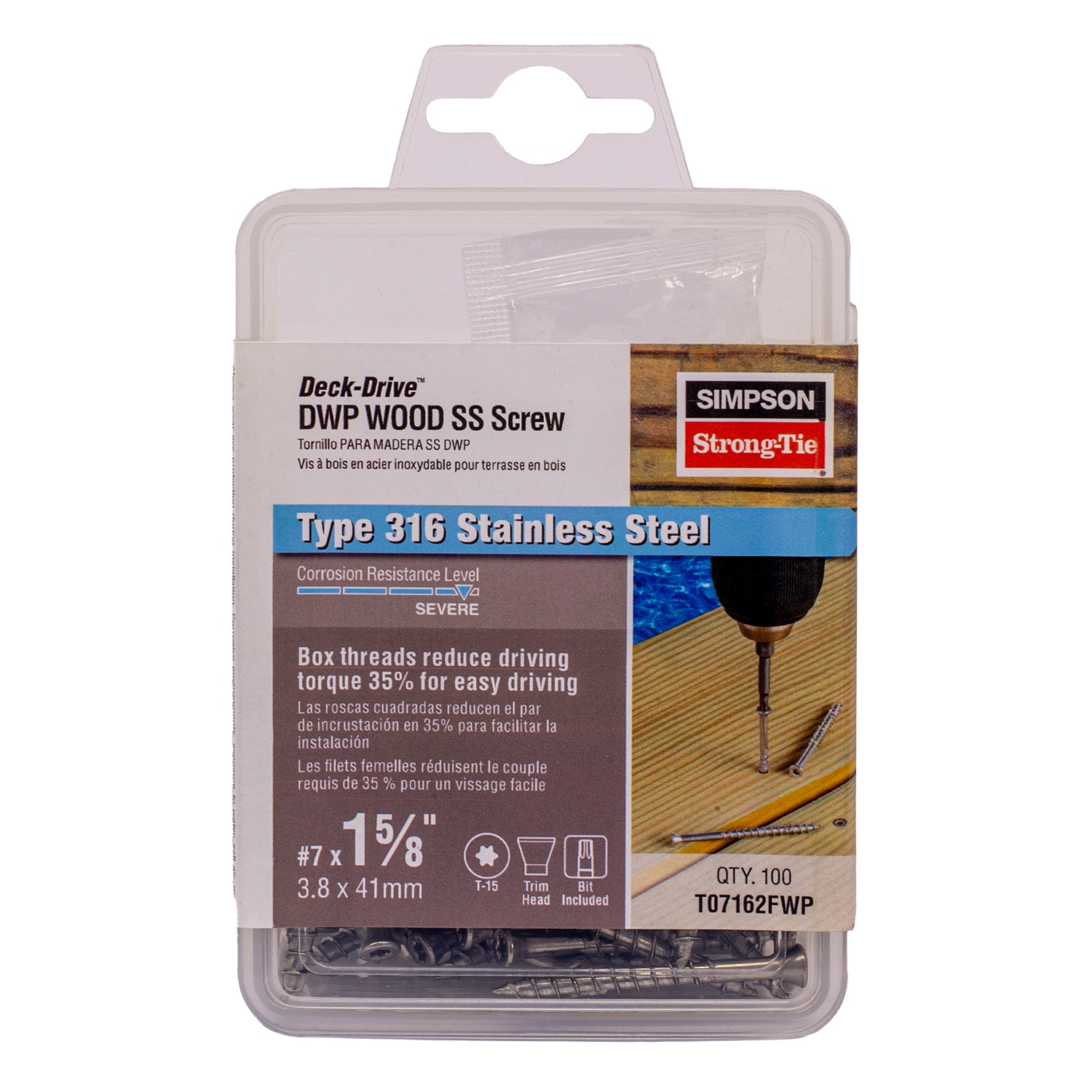The image depicts a plastic container of stainless steel wood screws, specifically the Deck Drive DWP Wood SS Screw from Simpson Strong-Tie. The container features a white top and a clear bottom through which some of the silver screws are visible. It also has a hook for store display. Encasing the container is a detailed cardboard sleeve, prominently bilingual, including French explanations. The sleeve describes the screws as Type 316 stainless steel with a "Severe" level of corrosion resistance. These screws are designed to reduce driving torque by 35% for easier driving, thanks to their boxed threads. They have a trim head and each screw measures 1-5/8 inches, or 3.8 x 41 millimeters. The package includes 100 screws and a bit. On the side of the sleeve, there's an illustration of an electric drill driving a screw into a plank of wood, providing a visual demonstration of their use.